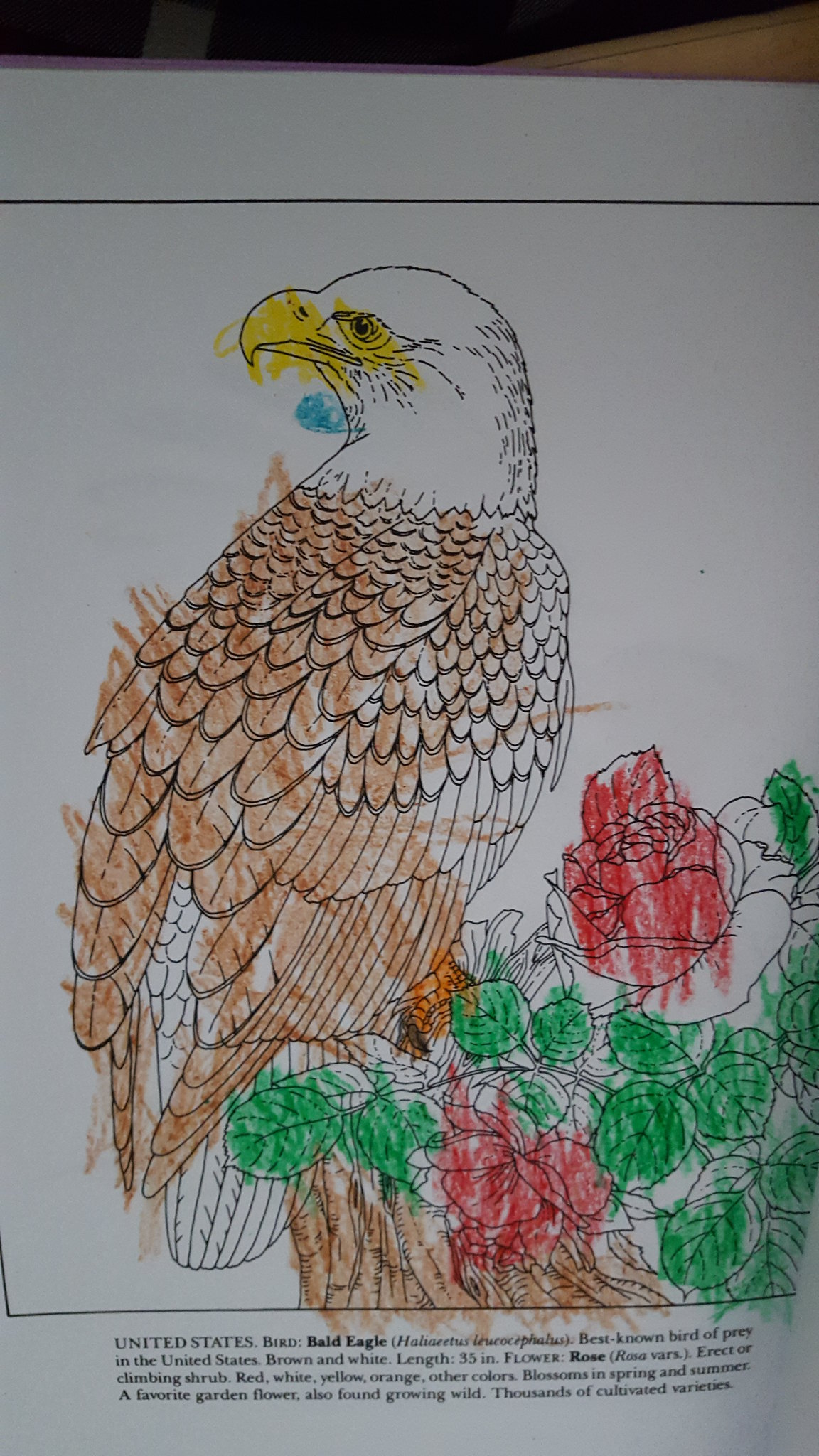This photograph captures a page from a coloring book resting on a brown desk with a bit of black in the background. Dominating the page is an illustration of a bald eagle, its back turned towards the viewer while its head faces left in profile. The eagle, outlined in black ink, stands perched on a rose bush in the lower right-hand corner. A caption beneath the eagle in small black font provides descriptive details and facts about the bird and the rose bush. The child who colored the page used crayons, although not within the lines. The eagle's feathers are primarily brown, with some portions left white. The beak and eyes are colored yellow, with a blue crayon mark on the neck. The rose bush features red roses and green leaves, with the branches colored the same brown as the eagle's wings.